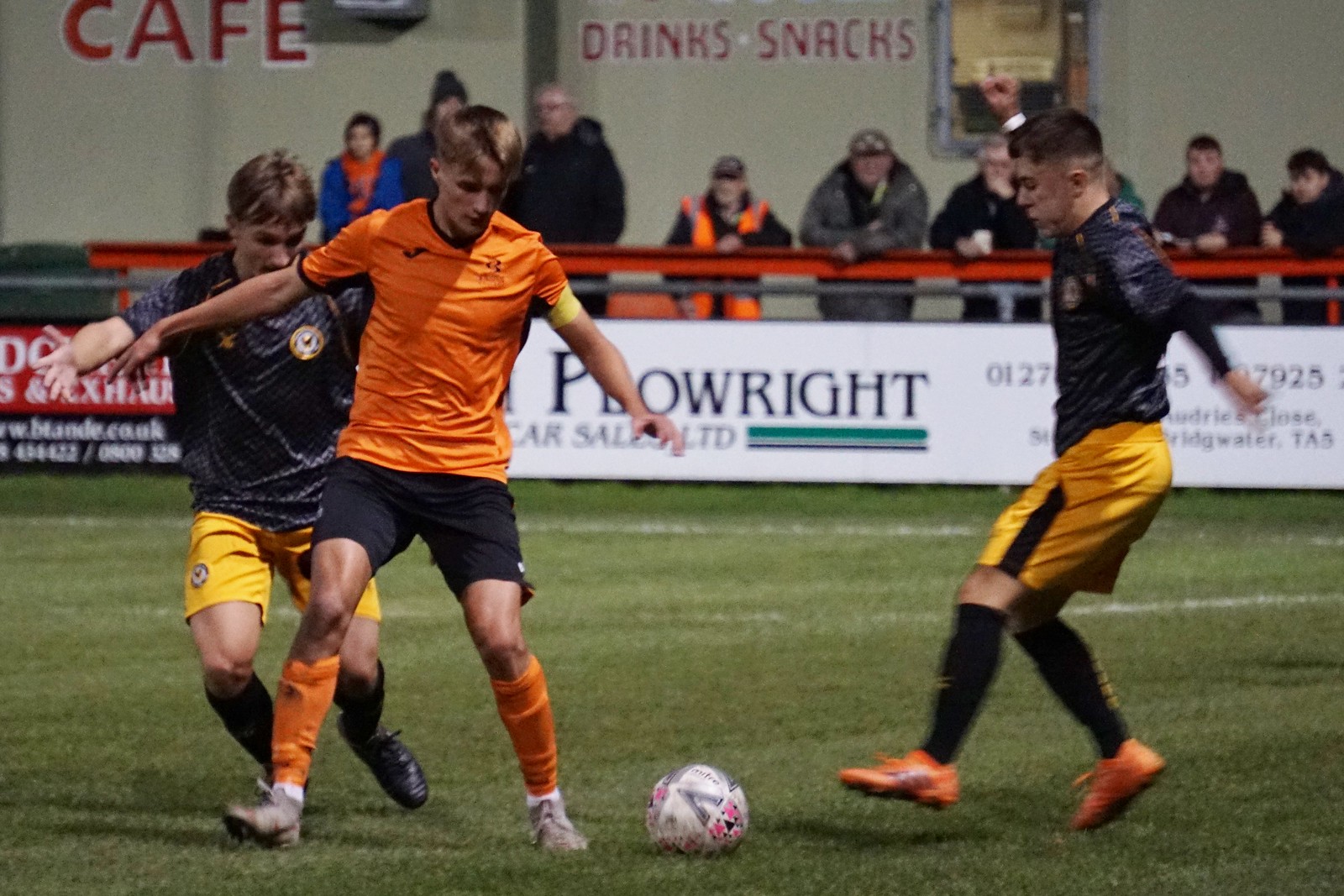In this detailed photograph, three soccer players are intensely focused on a white soccer ball with black and pink triangular designs, positioned at the feet of the center player in an orange jersey, black shorts, and orange socks. This player, with extended hands, appears ready to engage with the ball, which is at his left foot on the vibrant green pitch. To his left stands an opposition player in a black jersey and yellow shorts, while another opponent in identical team colors with orange shoes hovers to his right. Both players in black jerseys and yellow shorts mirror the center player's focus on the ball.

The scene is vibrant and dynamic, set outdoors on a well-maintained soccer field. Behind the players, spectators lean over a horizontal orange metal barrier, watching the action intently. This barrier separates the field from a background where sponsorship banners are prominently displayed. The fence features a white sign reading "Plow Right, Car Sales Limited" in dark print, along with another that advertises "Drinks, Snacks, Cafe" situated above the heads of about ten spectators. These onlookers, some actively engaging with the game, add to the atmosphere with their presence. The image captures a snapshot of riveting sports action, framed within the context of a lively and engaging soccer match.